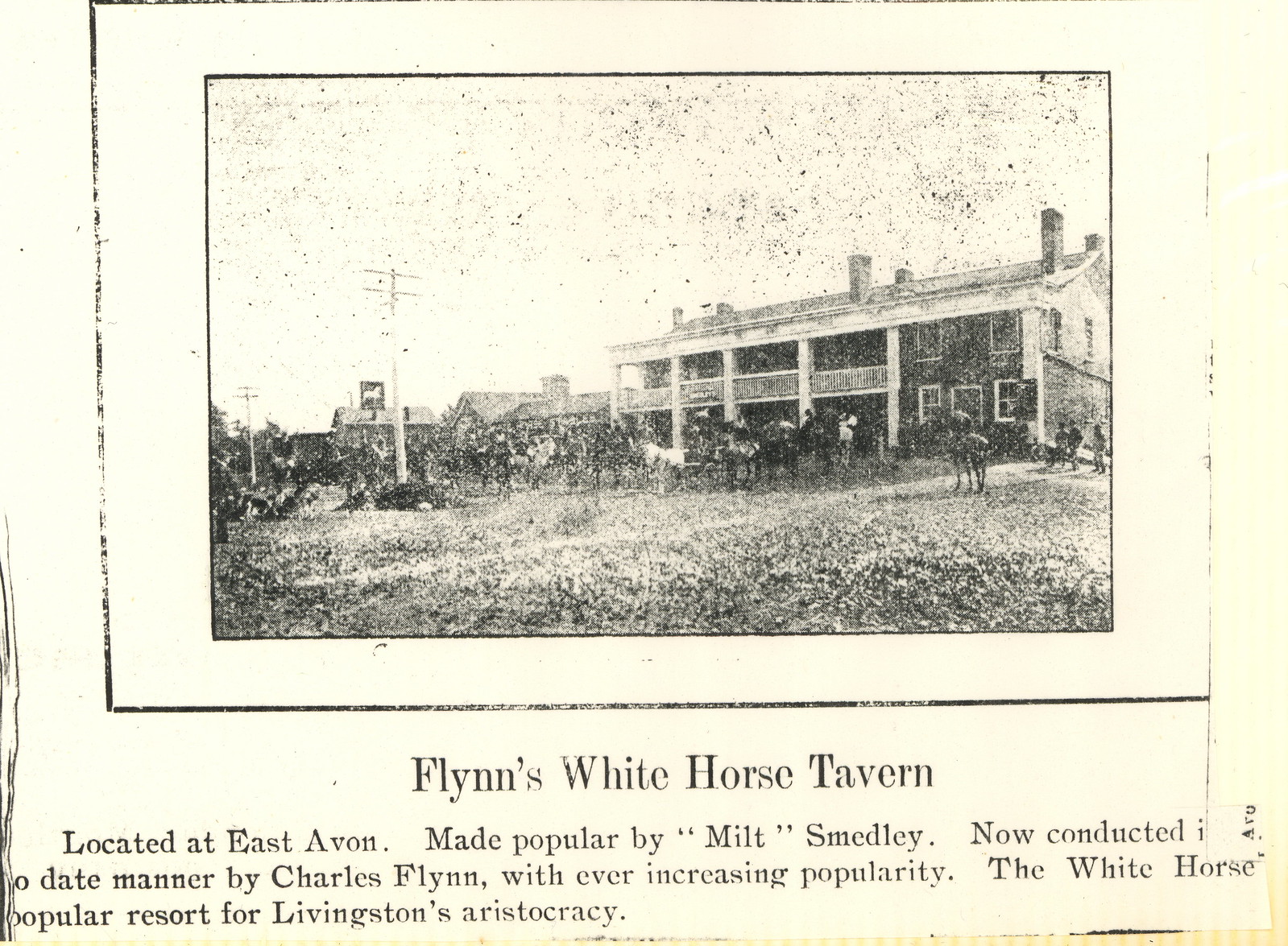In this black and white, newspaper-style image, we see a historic building identified as Flynn's White Horse Tavern, located in East Avon. The tavern, depicted in a detailed photograph, stands as a popular resort once frequented by Livingston's aristocracy. The multi-story structure features balconies on the left side, numerous windows, and is supported by five prominent pillars at the front. The building also has two or three chimneys atop its roof. In front of the tavern, there are several horses and men gathered, adding a lively touch to the scene. The street in front of the building appears to be dirt with patches of grass, and more buildings are visible further down the road on the left. Tall poles, likely telephone poles, line the street. The photograph is encased in a double-black rectangular outline, and below it, in bold black writing, it reads, "Flynn's White Horse Tavern." Additional smaller black print underneath mentions the tavern's popularity first under Milt Smedley and continued success with Charles Flynn. The scanned image captures a moment in time, preserving the cultural and historical significance of the once-popular establishment.